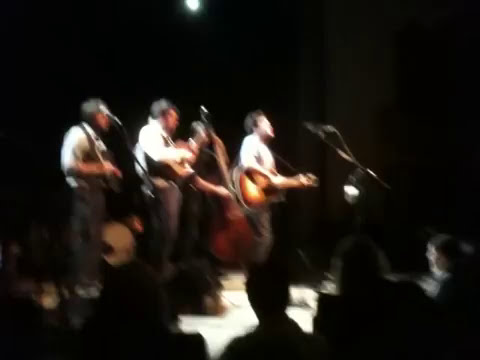In a dimly lit, possibly intimate setting reminiscent of a nightclub or outdoor dark stage, a band is performing, with the lighting casting down dramatically from above. The stage is populated by three main visible men, all wearing formal black and white attire. Off to the center left, one man appears to be wearing a hat and possibly suspenders, while holding a banjo. The middle man, dressed similarly in a white shirt, is playing a guitar or ukulele. The third man, on the right, is also holding a guitar and appears to be singing into a microphone. Only the arm of a fourth band member, behind the second musician, can be seen, indicating they are playing a large bass. The image is blurry, complicating distinct identification of instruments and finer details. In the foreground, silhouettes and outlines of an engaged audience are visible, suggesting they are seated close to the stage, focusing intently on the performance. The overall ambiance is shadowy, enhancing the intimate atmosphere of the scene.